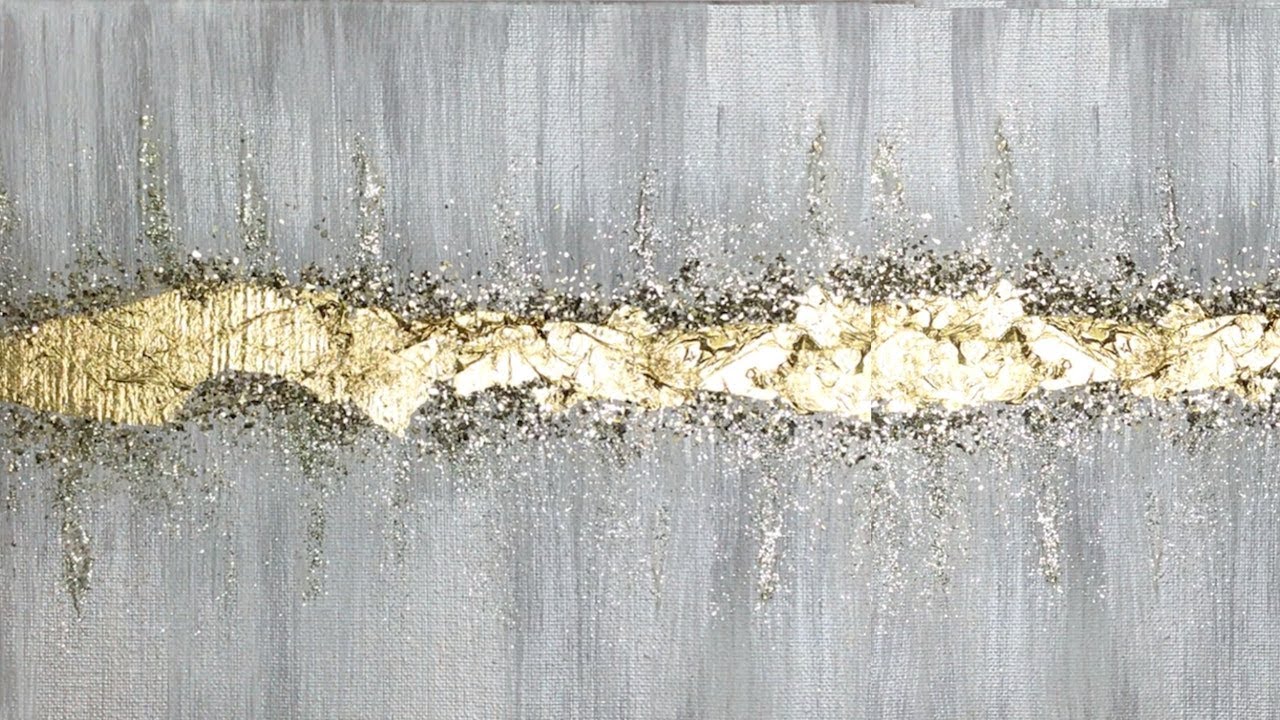This detailed close-up image centers on a predominantly gray, textured surface that seems to have been either damaged, sanded, or sawed into, extending horizontally across the frame. The texture shows variable shades of light and dark gray, contributing to a natural, somewhat weathered appearance. Through the middle runs a jagged, uneven fissure, irregular like a curvy river or lightning bolt, marked by a striking lack of uniformity. This fissure reveals a lighter, tan-colored layer beneath the gray surface, which gradually transitions to a nearly white color towards the right side. Along the edges of this jagged cut, there are scattered bits of debris, resembling sawdust or particles of dust, indicating recent agitation or disruption of the material. The fissure's exposed layer has a shiny, reflective quality that hints at a golden hue in some descriptions, adding a subtle highlight amidst the more somber tones. The overall effect is an abstract, textured landscape marked by natural patterns and an unorganized break, which adds an intriguing, almost artistic element to the image.